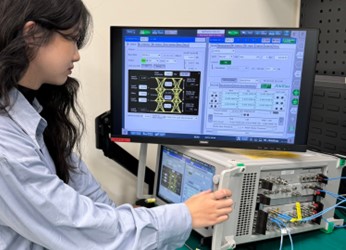The image depicts a young Asian woman with long black hair, dressed in a light blue, long-sleeved lab coat with a collar, suggesting she might be a nurse, an engineer, or a lab assistant in a scientific or medical setting. Positioned to the left of the frame, she is seen intently analyzing data on a large monitor that displays information in various colors including light blue, dark blue, green, yellow, and black, set against a cream-colored wall. Her right hand is placed on a complex piece of computer-like equipment beneath the monitor, which features multiple ports and an array of cables. This secondary device, which also has its own screen, indicates that she is engaged in a detailed and technical task, possibly involving scientific testing or calibration of medical apparatus.